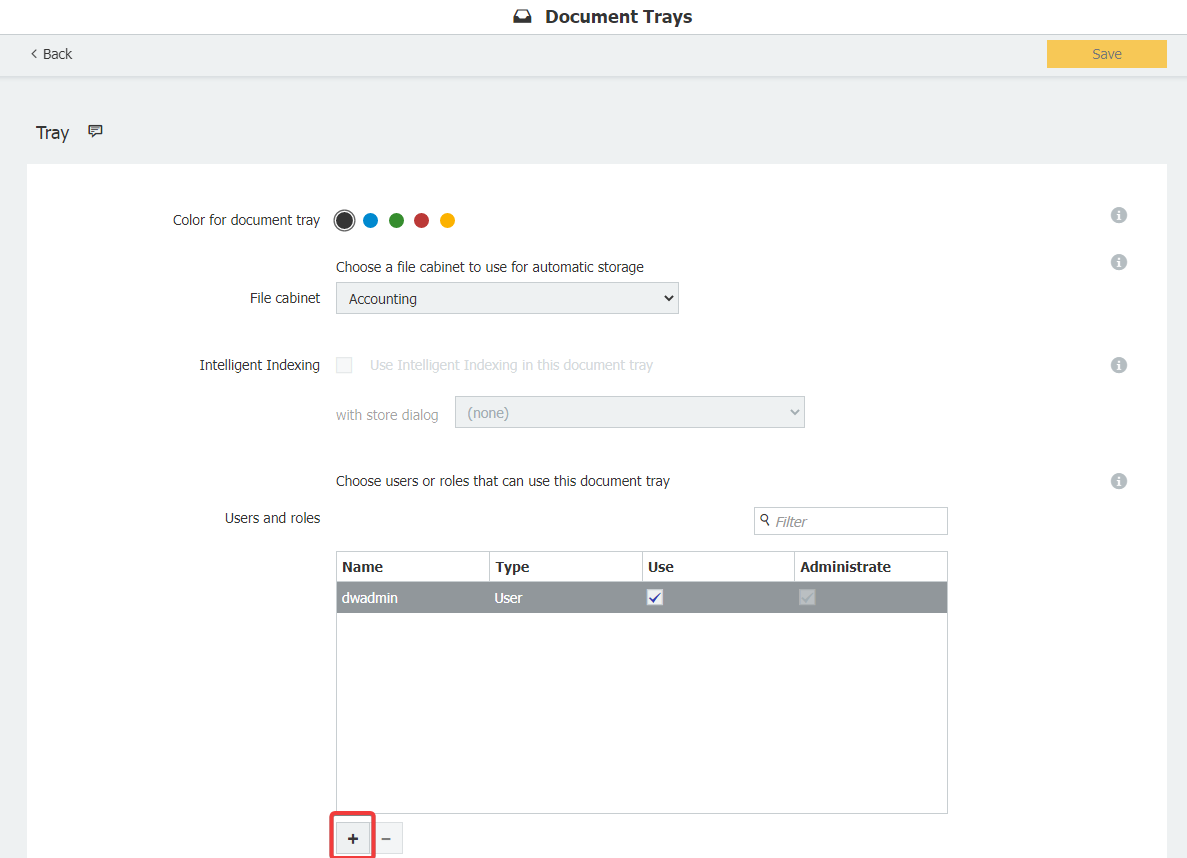In the image, the top section is shaded in gray. Above this gray area, the title "Document Trays" is prominently displayed. On the top left corner of the gray section, there's a back button, whereas on the top right, a vivid orange rectangle is labeled "Save." 

Below the gray area, on the left side, the word "Tray" is clearly written. Underneath this, set against a white background, the label "Color for Document Tray" is present. Accompanying this label are circles in different colors: a highlighted black circle, followed by blue, green, red, and orange circles.

Further down, there's an instruction that reads, "Choose a file cabinet to use for automatic storage." Directly below this, the term "File Cabinet" is situated to the left. Adjacent to it, a gray drop-down menu displays the option "The Accountant."

Below the drop-down menu, there's a section titled "Intelligent Indexing" with an unchecked box next to the label "Use Intelligent Indexing in the Document Tray for Store Dialog." A drop-down menu beneath this section is initially set to "None."

Continuing down, there's guidance to "Choose users or roles that can use this document tray," next to which the phrase "Users and Roles" is located. Beside it sits a search bar labeled "Filter," accompanied by a magnifying glass icon. Directly under the search bar, there's an empty box ready for input.